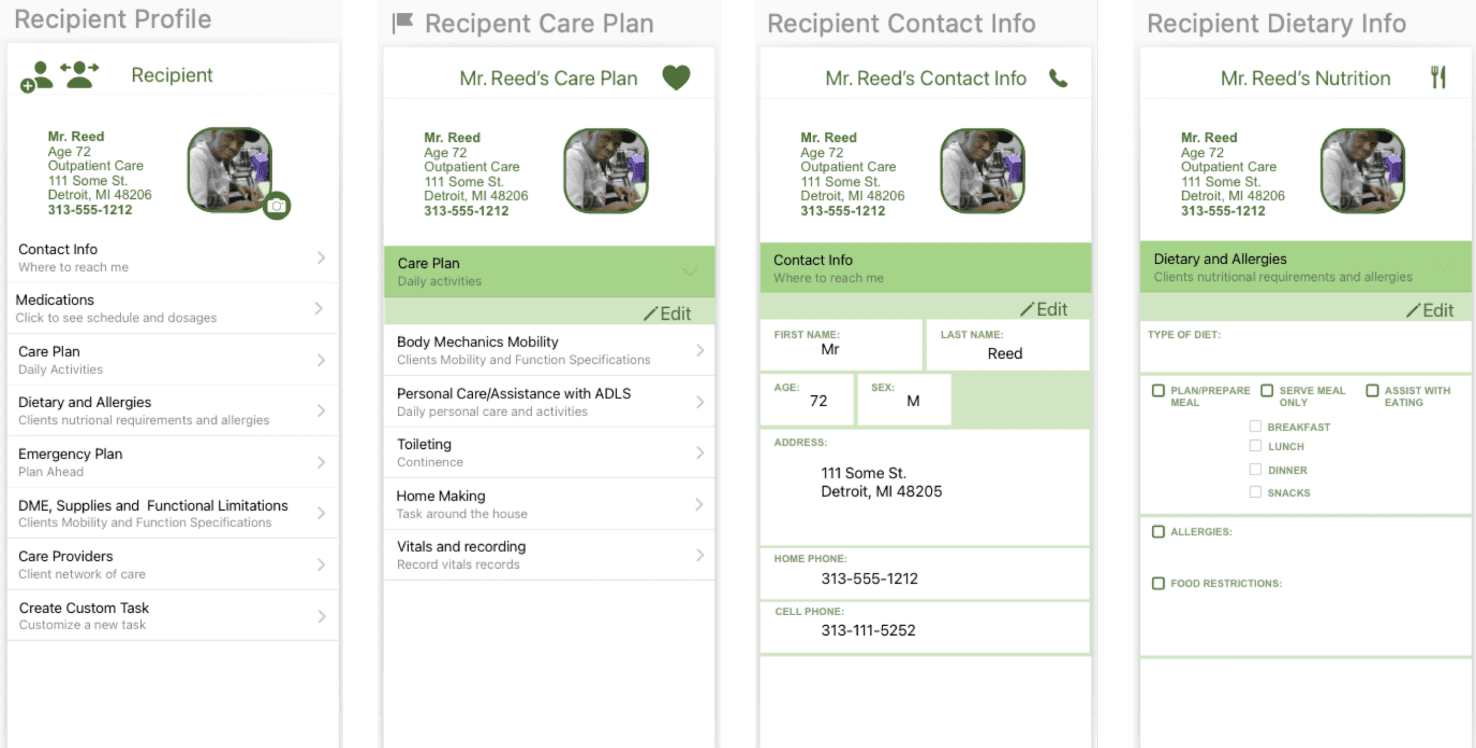The image is a collage of four smaller images focusing on the care details and contact information of Mr. Reed, a 72-year-old outpatient car recipient from Detroit, Michigan.

1. **Recipient Profile:**
   - A profile of Mr. Reed, including a square photo of an African American man.
   - Detailed contact information: Address: 111 Some Street, Detroit, MI 48206; Home Phone: 313-555-1212.
   - Sections highlighted:
     - Contact Info: Where to reach Mr. Reed.
     - Medications: Schedule and dosages.
     - Care Plan: Daily activities.
     - Dietary and Allergies: Nutritional requirements and allergies.
     - Emergency Plan: Contingency preparations.
     - DME Supplies and Functional Limitations: Mobility and function specifications.
     - Care Providers: Client’s network of caregivers.
     - Create Custom Task: Option to customize a new task.

2. **Care Plan:**
   - Reiterates Mr. Reed's profile details with the same photo.
   - Sections include:
     - Care Plan: Daily activities (with an edit option).
     - Body Mechanics & Mobility: Functional specifications.
     - Personal Care/Assistance with ADLs: Daily activities and personal care.
     - Toileting & Continence.
     - Homemaking: Tasks around the house.
     - Vitals & Recording: Vital records management.

3. **Contact Info:**
   - Detailed contact information for Mr. Reed is expanded:
     - First Name: Mr.
     - Last Name: Reed
     - Age: 72
     - Sex: Male
     - Address: 111 Some Street, Detroit, MI 48205.
     - Home Phone: 313-555-1212.
     - Cell Phone: 313-111-5252.
   - This section includes an edit option for updating contact information.

4. **Nutrition:**
   - Focuses on Mr. Reed's dietary needs and allergies.
   - Sections include:
     - Type of Diet (currently blank).
     - Options for meal planning, preparation, serving, and assistance with eating categorized into Breakfast, Lunch, Dinner, and Snacks (none of which are checked).
     - Allergies and Food Restrictions sections, both currently without any checks.

Each image provides a comprehensive set of details, presenting an organized approach to managing Mr. Reed's healthcare needs.